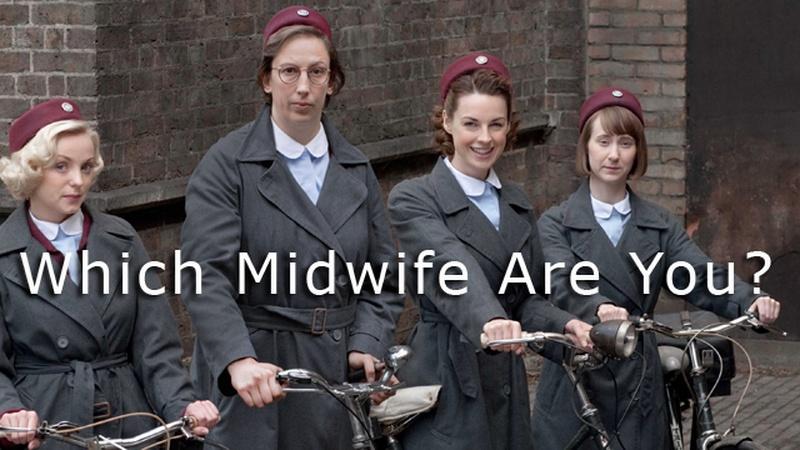This photograph captures four young to middle-aged women, all dressed identically in uniform, standing with their bicycles in front of a brick building. Each woman is outfitted in a light blue blouse under a cinched gray raincoat and wears a maroon beret featuring a circular pin. The text "Which midwife are you?" is prominently displayed in white lettering towards the lower middle section of the image. The women have neat, short hairstyles and all wear similar dark gray raincoats. The lady on the far left has blonde hair, while the others, including the tall woman second from the left with glasses, are brunettes. One of the bicycles, specifically the second from the right, is equipped with a light. They appear ready to make their rounds, serving as midwives.